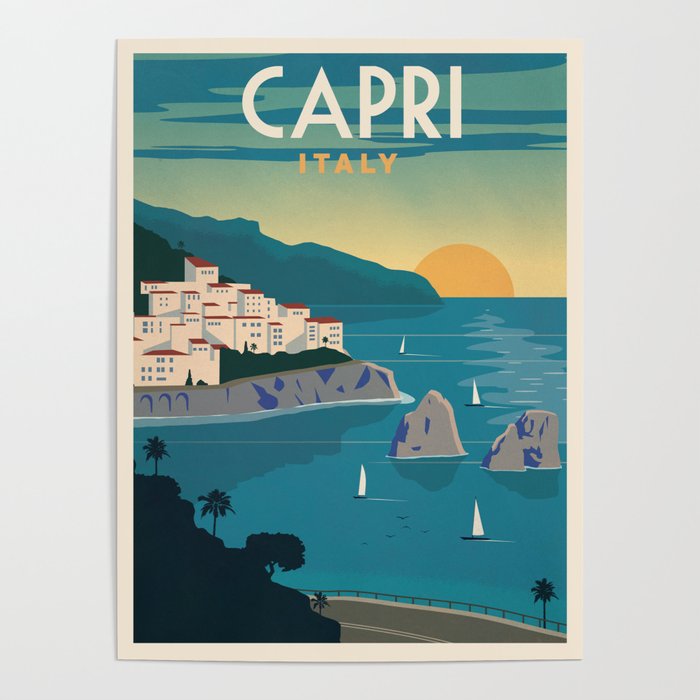This image is a postcard-style painting depicting a scenic view of Capri, Italy. It is framed by an off-white or beige border. At the top, the word "Capri" is written in white text, with "Italy" in smaller yellow letters underneath it. The artwork captures a picturesque landscape under a sun, likely during sunrise or sunset, casting a warm light across the scene. 

In the background, a mountain range emerges from the horizon, creating a dramatic backdrop. The right side features a prominent sun, half-submerged, hinting at either dawn or dusk. A peninsula adorned with charming white buildings and red or orange roofs extends into the blue-gray ocean. Several sailboats with white sails dot the water, amplifying the coastal charm.

Notable rock formations protrude from the sea, adding to the rugged beauty of the scene. In the foreground, silhouettes of palm trees and a nearby hill or mountain are visible, casting dark shadows. The scene also includes a road winding across the bottom of the image, tying the varied elements together. The sky features a gradient from light blue to yellow, with patches of gray-blue clouds, enhancing the atmospheric depth of the painting. Overall, the artwork is a simplified yet evocative rendition of the idyllic Capri coastline.